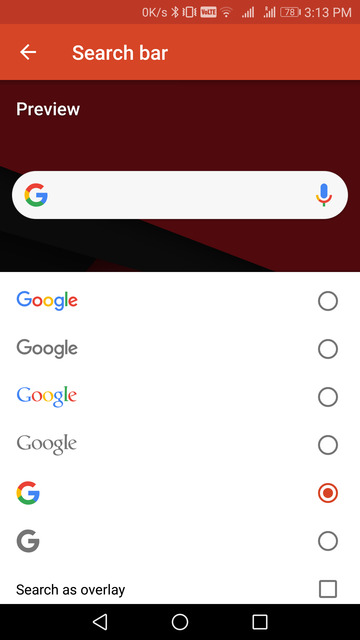This screenshot captures the interface of a cell phone screen with multiple layers of interface elements and icons displayed prominently. 

At the very top, a dark red status bar displays the time and various phone icons. Below this, a lighter red bar features a left-pointing arrow labeled "search bar." Directly beneath this, a black rectangle with the word "Preview" written in white is visible, followed by the Google search button, which includes a microphone icon for voice search.

Centered on the screen is the iconic Google logo, rendered in its traditional colors of blue, red, yellow, and green, adjacent to an empty black outline circle. Below this, the word "Google" appears in black with a similar outlined circle next to it. This is followed by various iterations of the Google logo, each presented in different fonts and color schemes.

Further down, a stylized "G" from the Google logo is displayed inside a red outlined circle with a red dot at its center. This is followed by another black "G" with an empty circle. Below these symbols, the phrase "Search as overlay" appears next to an empty square.

At the bottom of the screenshot is another black rectangle containing three white icons: a triangle pointing to the left, a circle, and a square. These icons likely represent navigation functions commonly found on Android devices.